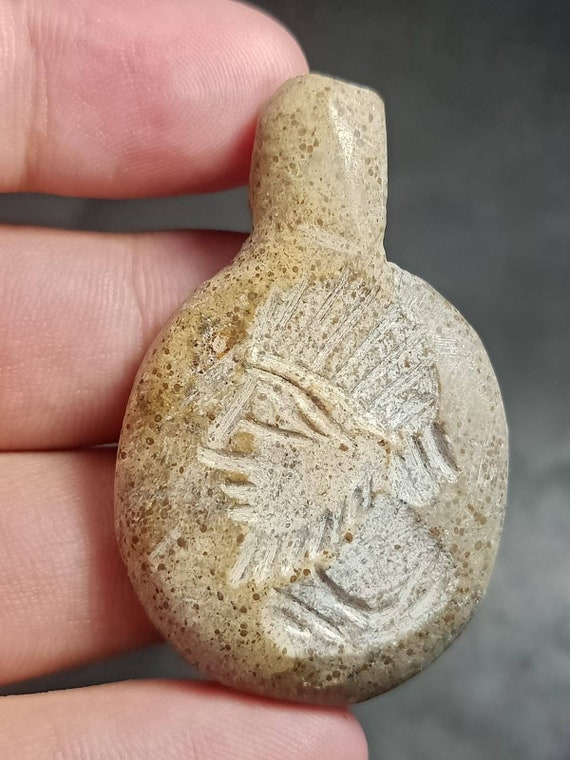The photo depicts a close-up of a left hand, with a lighter skin complexion, holding a very small, intricately carved beige stone or ceramic object. The object, resembling a tiny round speckled piece with a vertical tube at the top, fits snugly in the palm, with three and a half fingers visible around it. The front flat part of the object features a detailed, sanded-down engraving of a person's profile, showcasing large eyes, a pronounced nose, lips, and an ornate headdress that fans out above the face with hair flowing beneath. The overall clarity of the image is sharp, set against a gradient gray background, and the bright lighting enhances the object's delicate textures and carvings.